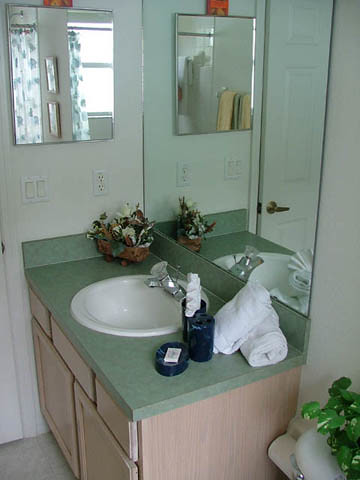The image showcases a bathroom with several distinct elements that enhance its cozy and functional atmosphere. 

In the top left corner, a small mirror reflects parts of the bathroom not visible directly in the image, including an open floral curtain and a closed floral shower or bath curtain. Below the mirror, there is a modern light switch with two rocker switches, alongside an electrical outlet.

A basket containing dried or synthetic flowers sits below this arrangement, adding a decorative touch to the space. The sink, made from a green, marbled material that resembles vinyl, is centrally featured. Above the sink is a larger mirror, providing ample reflection space. 

On the sink countertop, there are two liquid soap dispensers, a flat cake of hand soap, and a couple of neatly folded smaller towels. The vanity below the sink is made from light-colored wood, adding warmth to the otherwise white-walled bathroom.

In the lower corner of the image, part of the toilet can be seen with a plant on top, its green leaves providing a fresh, natural element to the bathroom's decor.